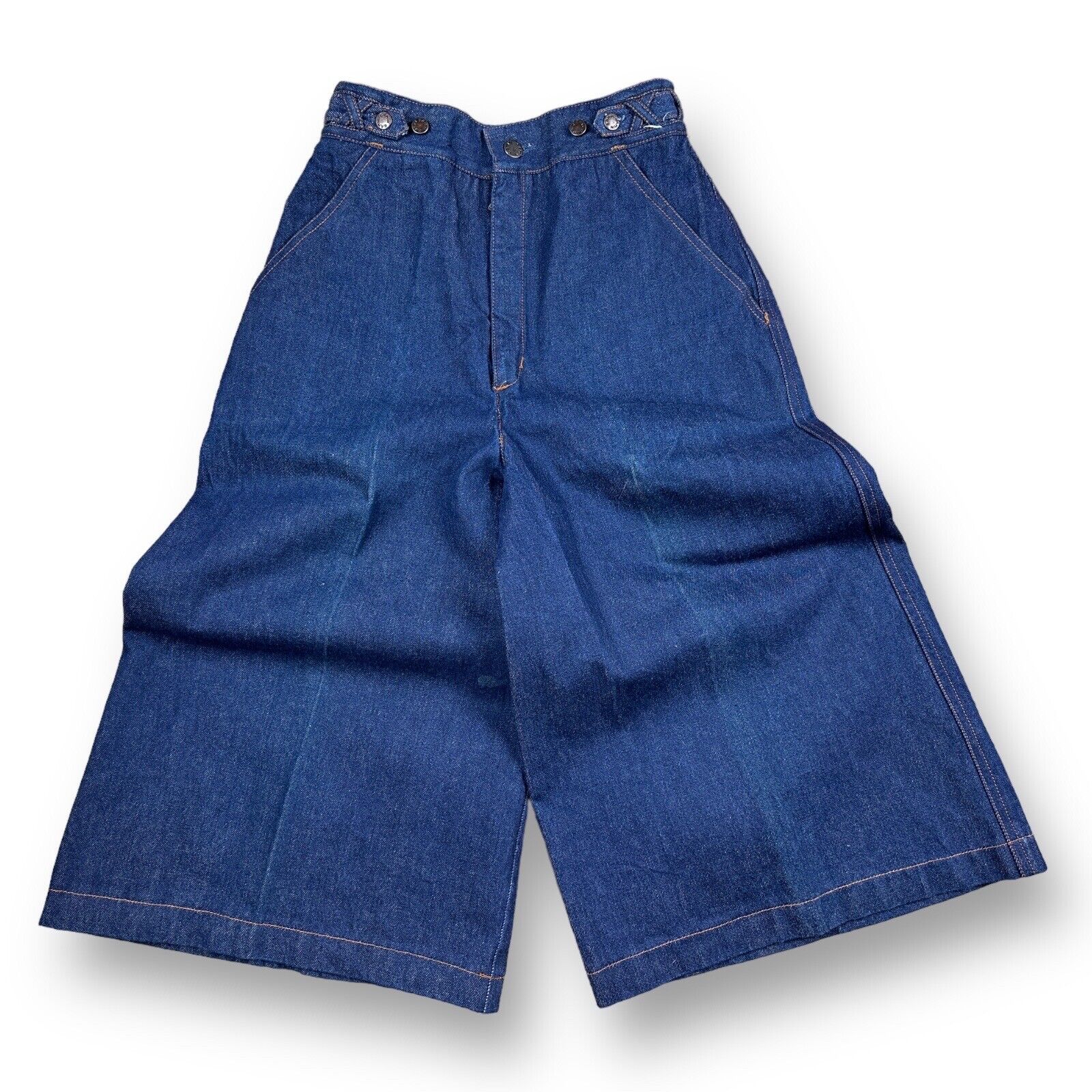This photograph shows a pair of blue denim shorts prominently displayed against a clean white background, likely intended for showcasing on a website or catalog. The shorts feature a very narrow waist, suggesting they are designed for a slim person, possibly a child or female. They are equipped with belt loops and are secured with gold button snaps at the top, highlighting their unique design.

The denim fabric is a darker, deeper blue, and the front of the shorts is characterized by pleats that lead down each side. Both sides of the waist have button straps, allowing for internal adjustment without needing a belt. The shorts possess two large pockets on either side, adding practicality to their design.

What stands out most about these shorts is the contrast in proportions: while the waist is quite narrow, the legs are exceptionally wide and baggy, giving them an almost skort-like appearance, particularly at the bottom. This exaggerated leg width creates a blocky, unconventional silhouette, making these shorts an intriguing and distinctive piece of clothing.